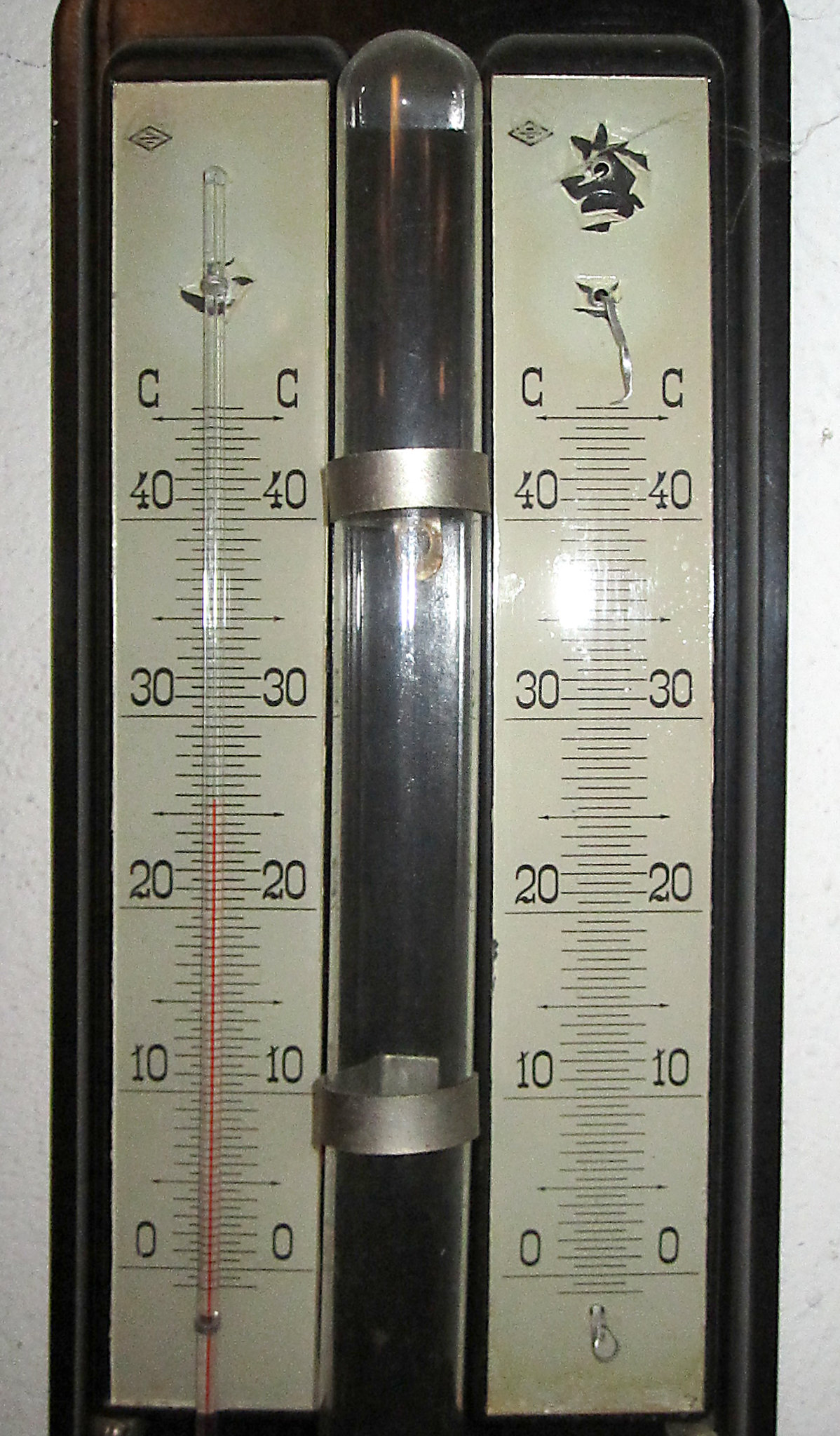The image depicts an antique thermometer featuring a mercury-based design, now considered obsolete due to the potential hazards of mercury exposure if the glass bulb were to break. Positioned on a wooden platform, the setup includes two thermometers side-by-side. One of the thermometers is missing its main component, while the other one indicates a temperature of approximately 26 degrees Celsius. 

In the upper right-hand corner of the image, there appears to be a curious element that resembles a picture of a witch, although it's unclear what it actually is. The thermometer is secured with metal brackets and accompanied by what might be a barometer in the center, though this isn't certain. The thermometer's setup includes old-fashioned lettering and possible metal elements or glued paper detailing. The thermometer that still remains intact is clamped with a small clasp, while the other is completely absent.